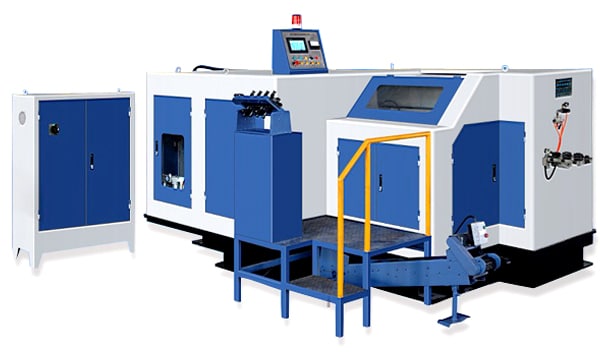The image showcases a complex piece of industrial machinery, characterized by its large, boxy structure adorned in white with blue panels and accents. The main body comprises two principal sections: a smaller, upright white cabinet with blue doors on the left, and a significantly larger piece of equipment on the right. This larger machinery features blue stairs that lead up to a platform equipped with a yellow handrail. Atop this platform, there's a control area with various panels, an access point with a viewing window, and an operational keypad complete with buttons, a small LED screen, and what appears to be a flashing red light indicating an error state. Additionally, there are fittings on the right-hand side that seem to be for plumbing supplies into the machine. Although its exact function remains unclear, the lack of exposed moving parts and detailed internal workings suggest a sophisticated, self-contained process, possibly resembling the operations of a 3D printer, water jet cutter, or industrial lathe.